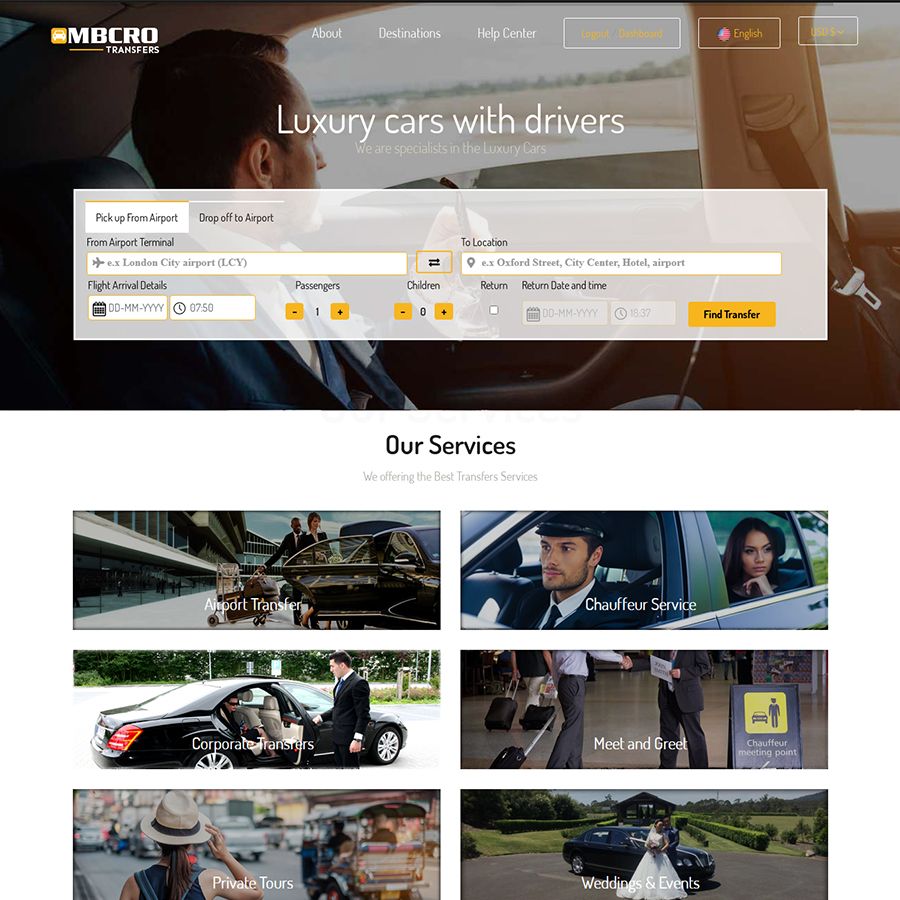In the top left corner of the image, the text "MPCRO Transfers" is prominently displayed in white against a vibrant yellow background, accompanied by an image of a sleek car. Above, several navigation tabs are visible, including "About," "Destination," and "Help Center." On the top right, there are three transparent buttons labeled in yellow: "Logout," "Dashboard," "English," and "US."

At the center of the image, a bold headline declares "Luxury Cars with Drivers." The subtext proudly states, "We are specialists in the luxury cars." Beneath this, a detailed form is provided for booking transfers, with fields for "Pick up from airport," "Drop off to airport," "From airport terminal," "London City Airport," "Flight arrival," "Date and Time," "Number of passengers," "Number of children," "Location," and "Return date." An orange button labeled "Find Transfer" is located at the bottom right of this section.

The background features a sophisticated image of a man wearing a suit, seated in the back of a car with the window slightly open, as the car travels to the right. At the bottom of the image, against a white background, the text "Our Service" stands out in black. This section outlines the services offered, arranged in two columns of three. On the left, the services listed are "Airport Transfer," "Corporate Transfer," and "Private Tours." On the right, they are "Chauffeur Service," "Meet and Greet," and "Wedding and Events."

The overall design combines a modern aesthetic with a high level of detail, emphasizing the luxurious and personalized nature of the transfer services provided by MPCRO.